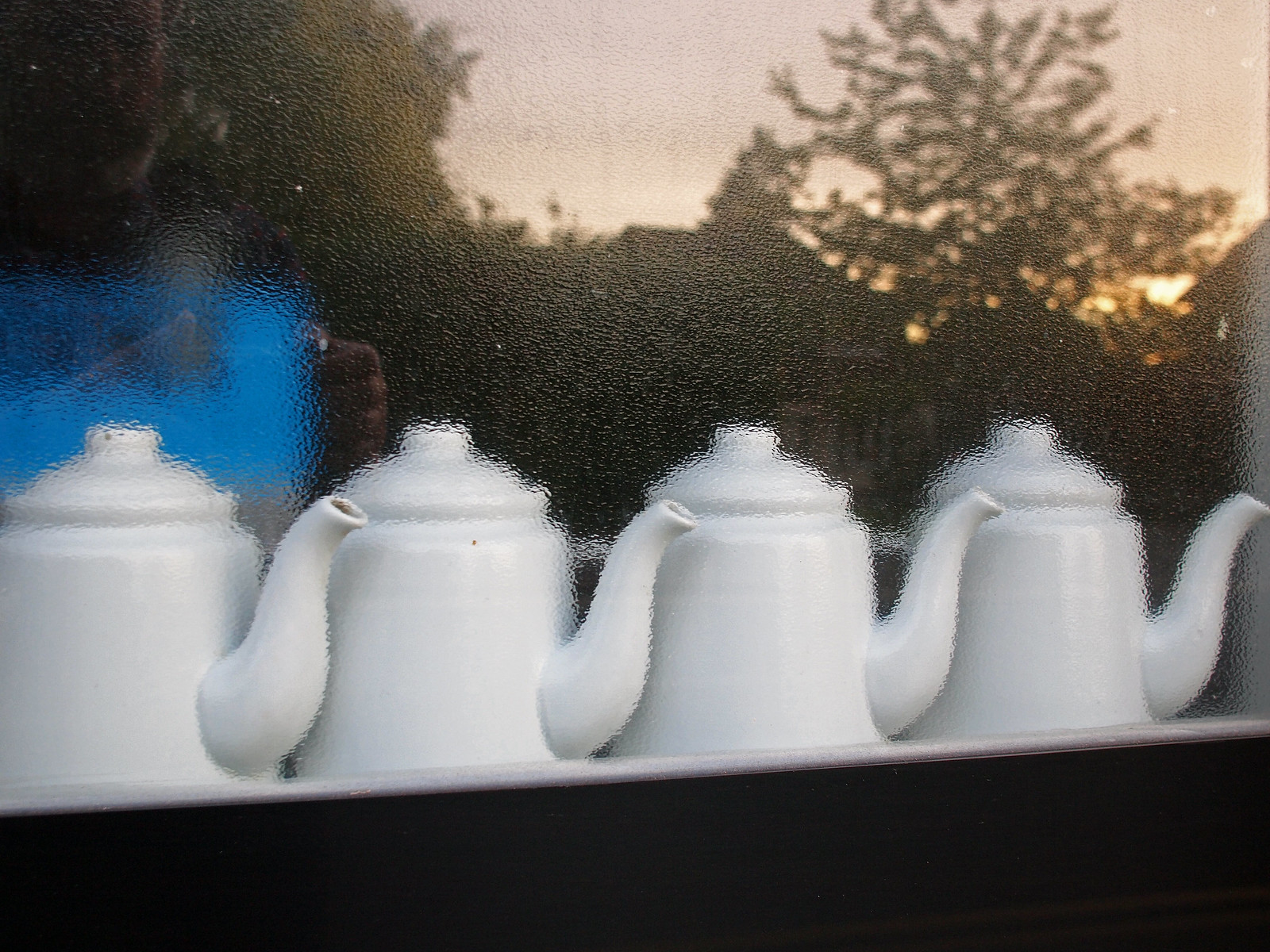The image, either a blurry photograph or a painting, depicts four white enamel teapots lined up in a row from left to right, viewed through a textured, bumpy glass window that distorts the scene. Each teapot is positioned with its spout facing to the right. The background reveals a sunset sky tinged with faint pink, purple, and yellow-orange hues. Above the teapots, the reflection shows the silhouettes of trees and house-like structures, with shadows emphasizing the depth. The upper left corner of the window features ripples, possibly from steam collecting, adding to the overall dreamy, surreal effect of the image.